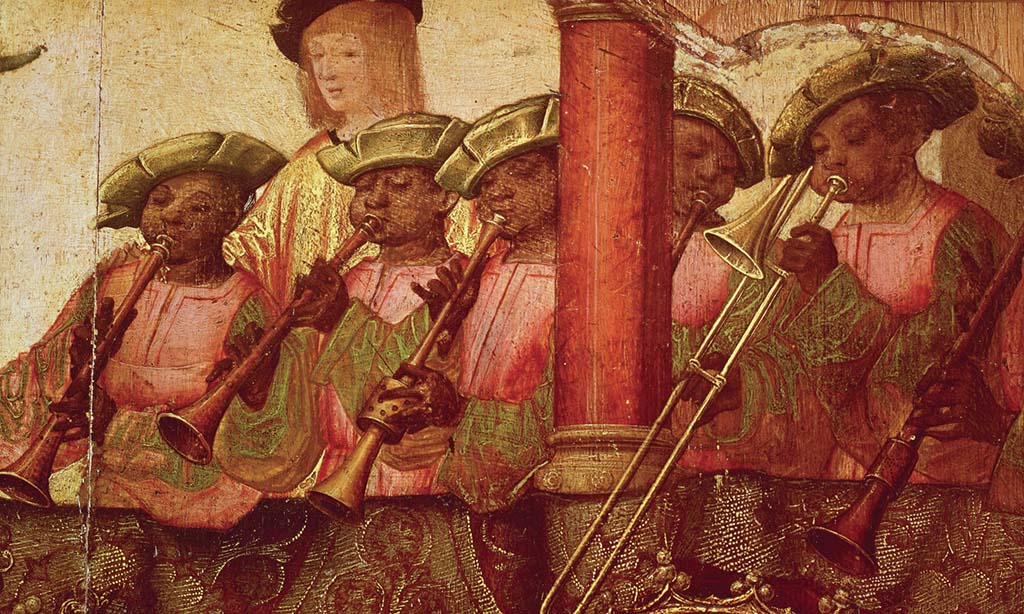This detailed section from an old, faded oil painting depicts a group of five children standing in a row, each playing various musical instruments, including trumpets, flutes, and trombones. The children are garbed in matching red and green robes with green hats, though some descriptions suggest variations like pink robes with tan sleeves, indicating possible wear and aging of the painting. Dominating the middle of the composition is a vertical red pillar, partially obscuring the faces of two children. Their skin tones vary, with some descriptions noting dark-skinned children, while one identifies a taller, white woman in the background. This woman, adorned in a gold dress with blonde hair and a black hat, watches over the children. The background of the painting is primarily gold, adding to the medieval aesthetic. Evidence of the painting's age includes visible cracks, peeling paint, and folded marks that disrupt the image, but its classic craftsmanship remains evident.